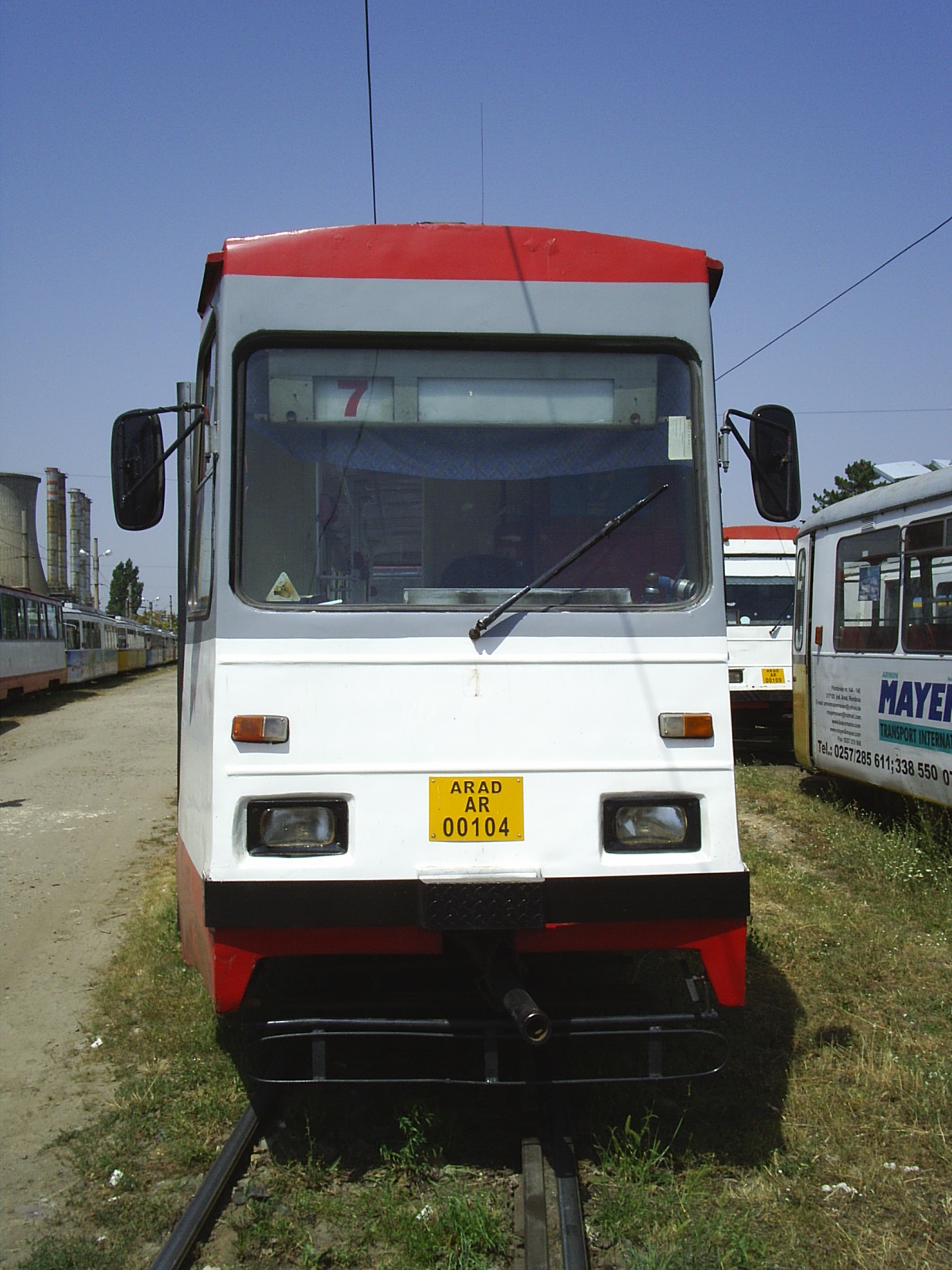This detailed full-color photograph captures an outdoor scene on a sunny day with a clear sky. At the center, there's a distinctive rail bus or trolley, which has a unique appearance combining features of both buses and trains. This vehicle is positioned on a grassy track, indicating it may have been stationary for a while. It has a white body with a red roof and a red bottom, adorned with a small yellow license plate that reads "ARAD AR 00104." The trolley features a large front window with a single windshield wiper and two rear-view mirrors on either side. A visible number "7" indicates it might be route number seven. Flanking the main rail bus are two other similar vehicles. To the left of the image, some buildings and possibly a road can be seen, contributing to the impression that this is a bus or trolley depot. The foreground shows a mix of pavement and tracks, while the sky above is cloudless, enhancing the bright, sunny ambiance of the scene.